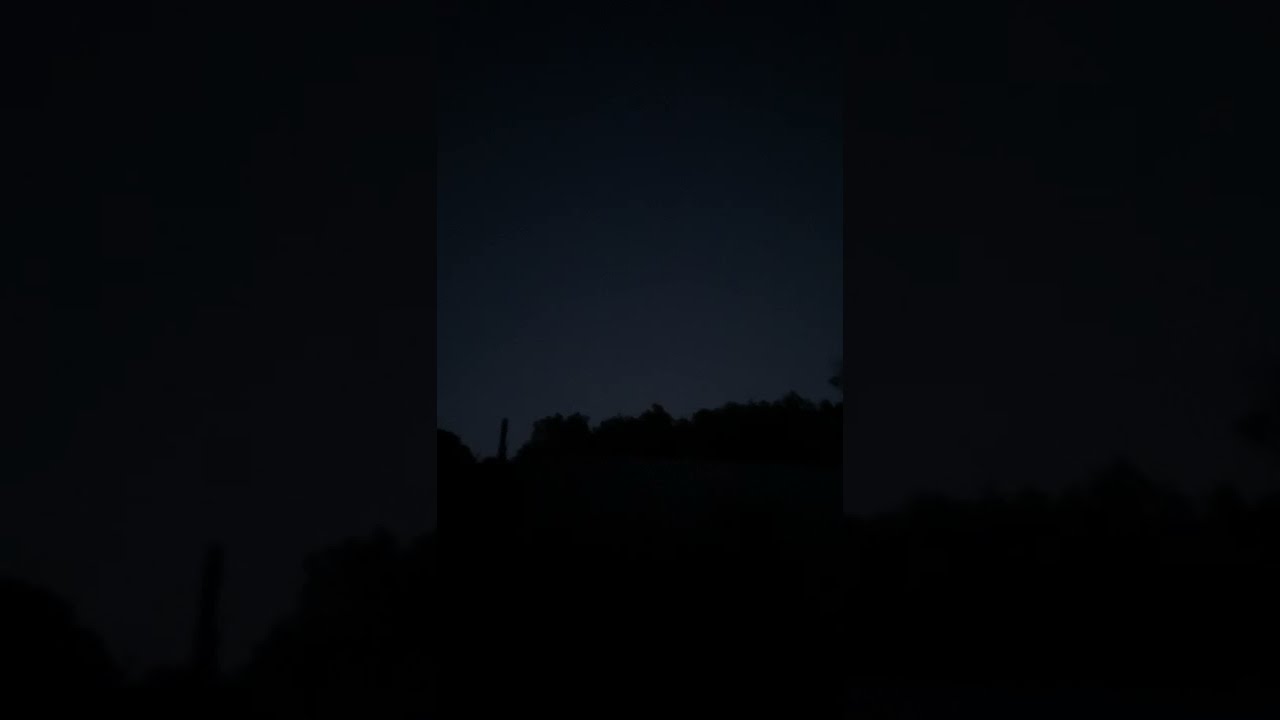The image in question appears to be a small icon or thumbnail that typically indicates an image unable to load. The icon is a tiny square with a dog-eared upper right corner and a white circle on a blue background in the upper left corner. The lower left corner seems to depict something green, possibly a mountain. Diagonally across the image, a white bar extends from the bottom center to the right center edge.

The main image itself is a dark, nighttime outdoor photograph primarily in black and gray tones. The bottom portion of the photograph shows the serrated tops of treetops with an object, possibly a rectangular column, protruding vertically among them. Above this section, the sky transitions from a lighter to a darker blue as it nears the top. The photograph features wide borders on both the left and right sides. These borders are composed of enlarged and grayed-out elements from the main photograph, making the image appear even darker but with some distinguishable lighter gray areas within the borders. The style of the photograph is realistic, capturing a serene yet shadowy nighttime woodland scene.